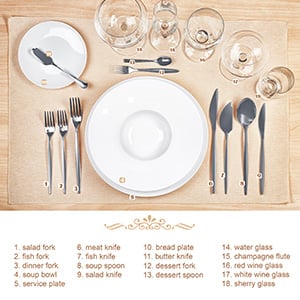This image depicts a detailed diagram of a formal place setting, meticulously arranged on a beige placemat atop a light brown wooden table. The layout includes an assortment of utensils, plates, and glasses, each carefully labeled. Starting from the top left corner, there's a small bread plate with a butter knife. Moving down to the center, there's a service plate with a soup bowl placed on top. On the left side of the service plate, the utensils are arranged in the following order: a salad fork, a fish fork, and a dinner fork. On the right side, the sequence is a meat knife, a fish knife, a soup spoon, and a salad knife. Above the service plate, there are a dessert fork and a dessert spoon. Directly above these, there's a water glass, followed by a champagne flute to the right, then a red wine glass, a white wine glass, and finally, a sherry glass. The image also features a numbered list from 1 to 18 below the place setting, identifying each item explicitly, enhancing its use as a guide for setting a formal dining arrangement.